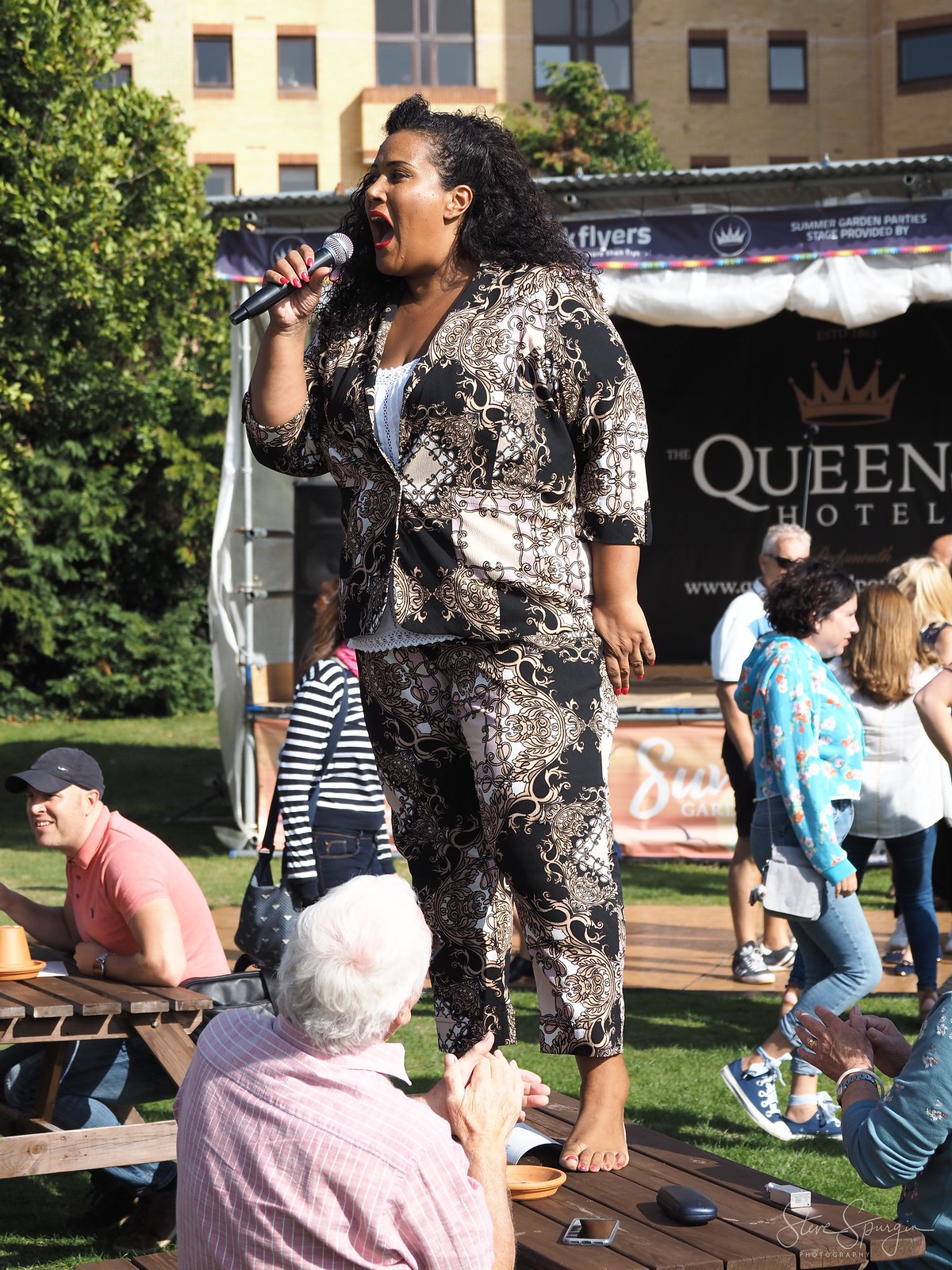In a lively mid-afternoon outdoor setting, an African American woman stands center stage on a picnic table, passionately singing into a black and silver microphone. She dons a striking ensemble consisting of a black, white, and gray printed jacket over a white blouse, paired with matching pants, and she is barefoot. Her long, curly black hair cascades over her shoulders, and her red lipstick adds a vibrant touch to her energetic performance. The woman is angled to the left in a three-quarter profile as she captivates her sparse audience predominantly comprising Caucasians.

Directly in front of her, a white-haired man clad in a pink short-sleeved shirt sits at the picnic table, clapping rhythmically in clear enjoyment. To her left, another seated Caucasian man in a red t-shirt and black baseball cap watches, his arm resting casually on the table. In the background, a group of people, some standing and others walking by, seem largely undisturbed by the performance. A few more attendees are clapping enthusiastically.

Behind the singer, a banner with bold white letters reads "Queen Hotel," partially obscured by the audience, with a multi-story building and a line of green leafy trees in the distance completing the park-like scene. The reflection of the sun and the relaxed atmosphere suggest a bustling yet joyful afternoon centered around the woman's dynamic performance.